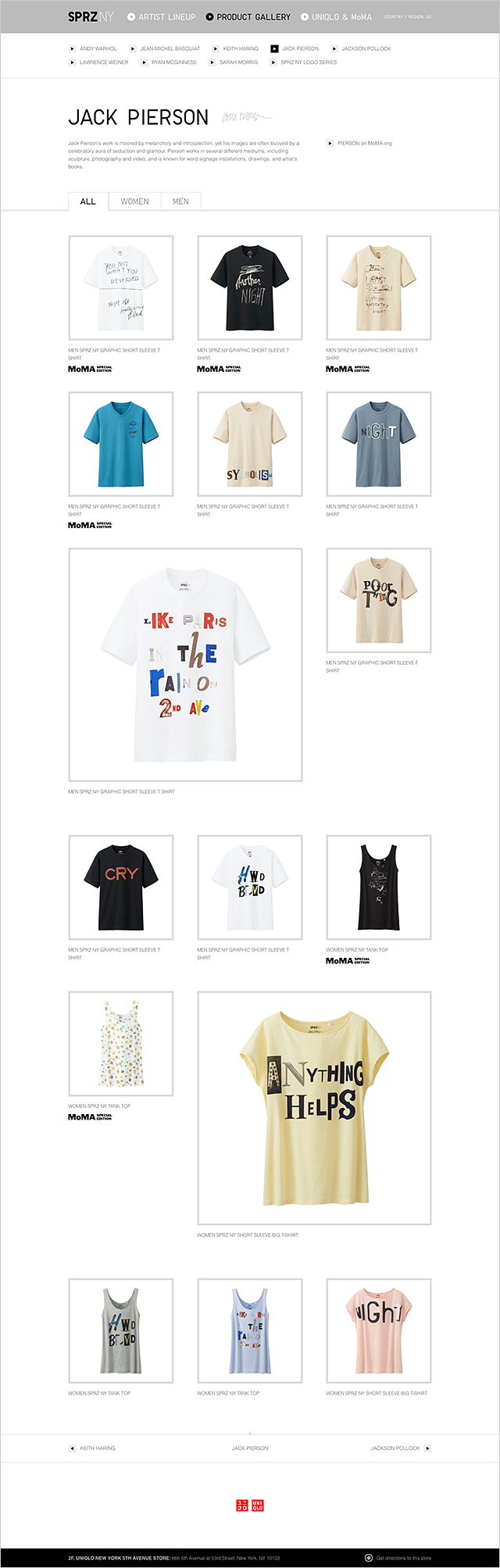This image is a screenshot taken from a shopping website displayed on a phone, characterized by its rectangular shape. At the top, there is a gray border running horizontally, about an inch from the left edge. Within this border, the text "SPRZ" is prominently displayed in all capital letters in black. Adjacent to it, in a smaller white font, is "NY," followed by a white circle containing a gray arrow. The text "artist lineup" appears in white next to a black circle with a white arrow. Moving to the right, the label "product gallery" is housed in a black color, succeeded by another white circle with a gray arrow. The term "UNIQLO and MoMA" is presented in white, and below that, small lettering denotes "country/region."

Beneath the gray border, the background transitions to white. There are small squares containing black arrows, aligned in pairs across several rows: two pairs on the left and two pairs on the right. Following these is a black square with gray detailing and a gray square with a black arrow underneath it. Positioned further right is another section with names of companies. The highlighted selection in black, indicating it has been clicked, is "Jack Pearson." Underneath Jack Pearson’s name, displayed in large all capital black letters, are three lines of detailed information.

Below this section, there are navigation tabs labeled "all," "women," and "men," with "all" being selected. This section features images of t-shirts arranged in a grid. The top row displays three t-shirts: one white and black with a tan hue, followed by explanatory text below each. The subsequent row features a blue t-shirt, a white t-shirt, and a gray t-shirt. Moving down, a larger square shows a white t-shirt and a smaller square with a tan t-shirt. Further rows include a black t-shirt, a white t-shirt, another black t-shirt, a polka-dotted t-shirt, a large tan t-shirt, and three more t-shirts at the bottom, variously colored.